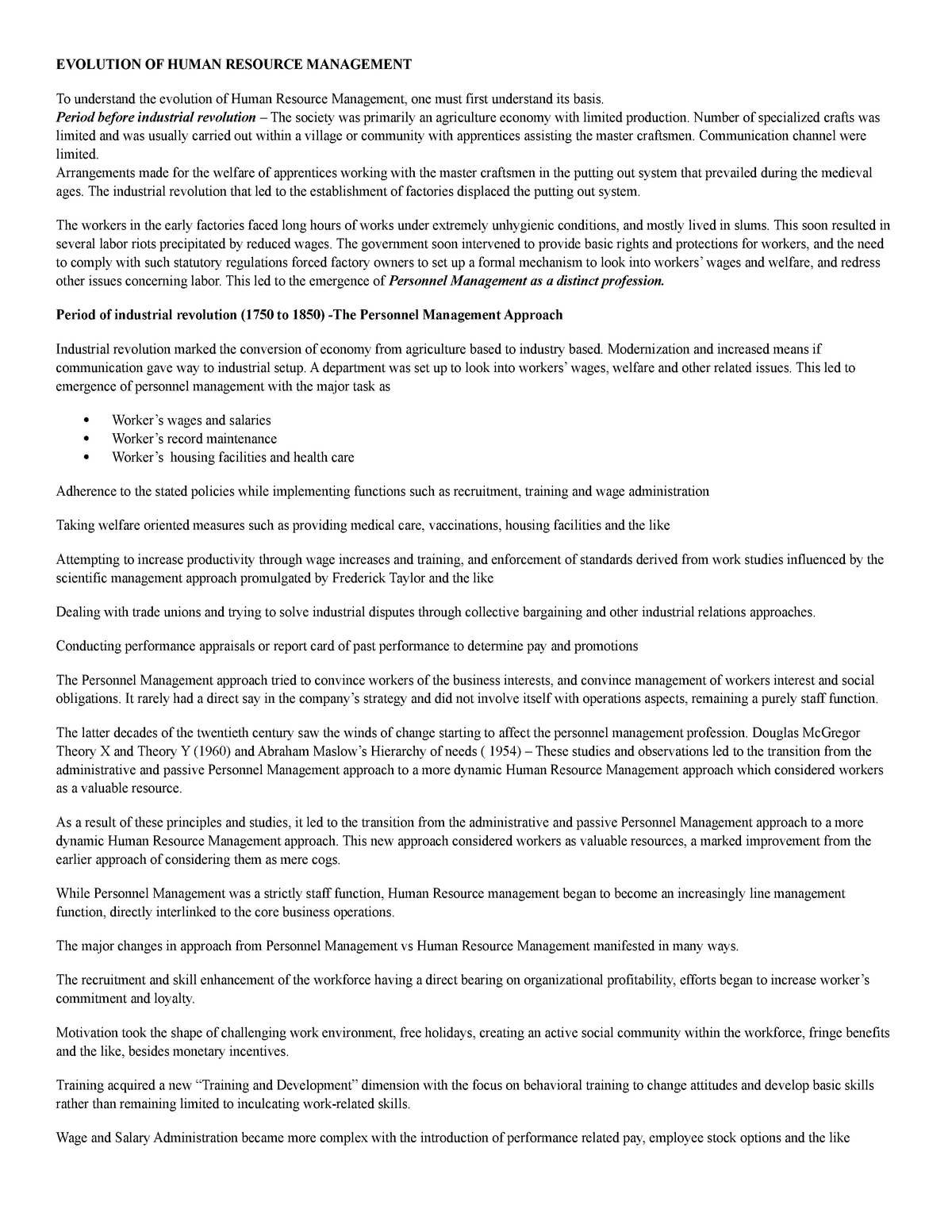Screenshot of an article or research paper detailing the historical context of human resource management. The document features a bold headline that reads "Evolution of Human Resource Management." It begins by emphasizing the need to understand the foundations of human resource management, which date back to the period before the Industrial Revolution. During this time, society was predominantly based on an agricultural economy with limited production capabilities. Specialization in various crafts was minimal, and these were usually performed within village or community settings, where apprentices worked under master craftsmen. Communication channels were constrained, and specific arrangements were made to support the welfare of apprentices. These arrangements were part of what was known as the putting-out system, which was prevalent during the medieval ages.